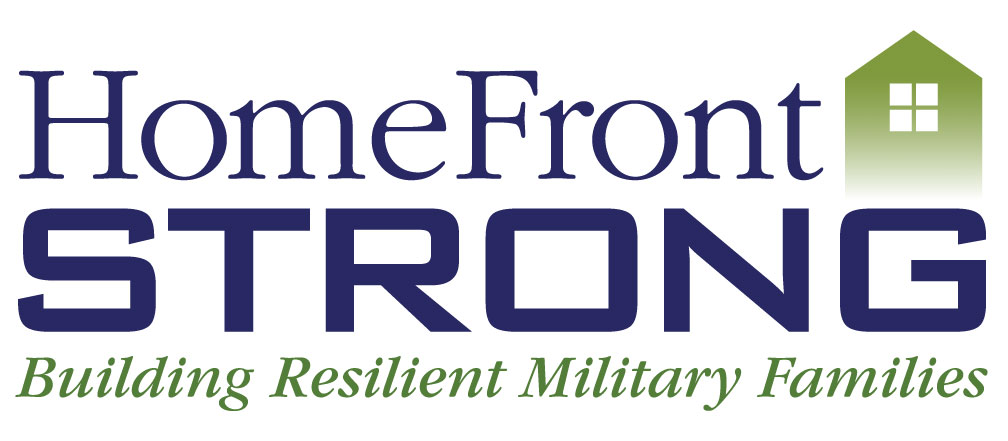The image features a predominantly white background with the word "Homefront" at the top in bold blue text. Directly beneath "Homefront" is the word "Strong," also in bold blue and capital letters. To the right of these words is a simple, green-colored rendering of a house with a pointed roof, a window with four panes, and no additional details. Below "Strong," in italicized green text, are the words "Building Resilient Military Families," depicting a focus on supporting military families. The clear and structured design suggests it could serve as a header for a website or a sign, emphasizing strength, resilience, and support for military families.